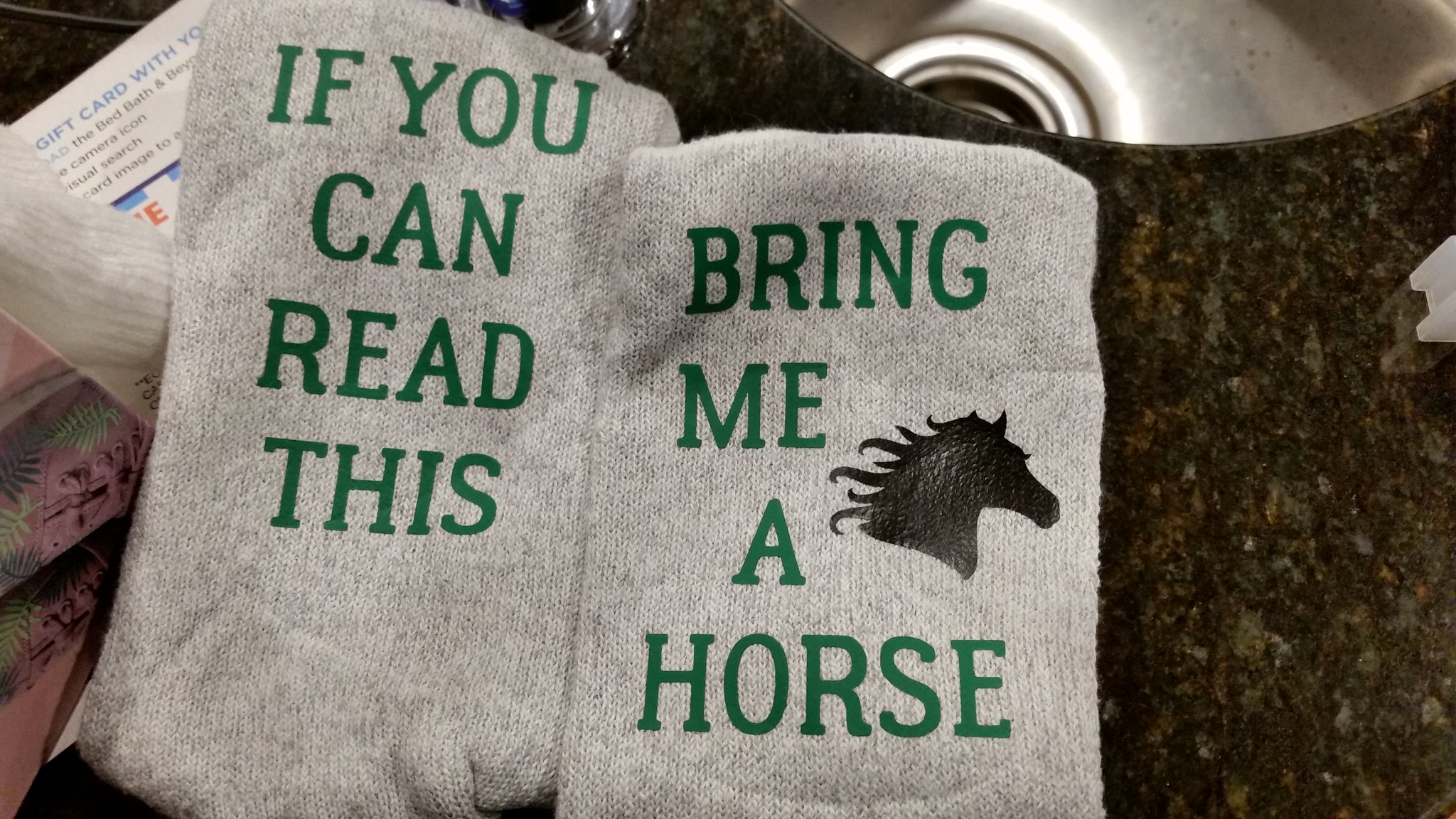This image showcases a pair of gray socks with green lettering placed on a black granite kitchen countertop. The left sock reads "If you can read this," while the right sock says "Bring me a horse," and features a black silhouette of a horse's head with a wavy mane. In the upper right corner, part of a metal kitchen sink is visible, along with the base of a faucet. To the left of the socks, there's a partially obscure paper or flyer with phrases like "gift card with your," "Bed Bath & Beyond," and "visual search card image." Additionally, there are some indistinct pink items with green leaves and possibly maroon drawings near the socks.